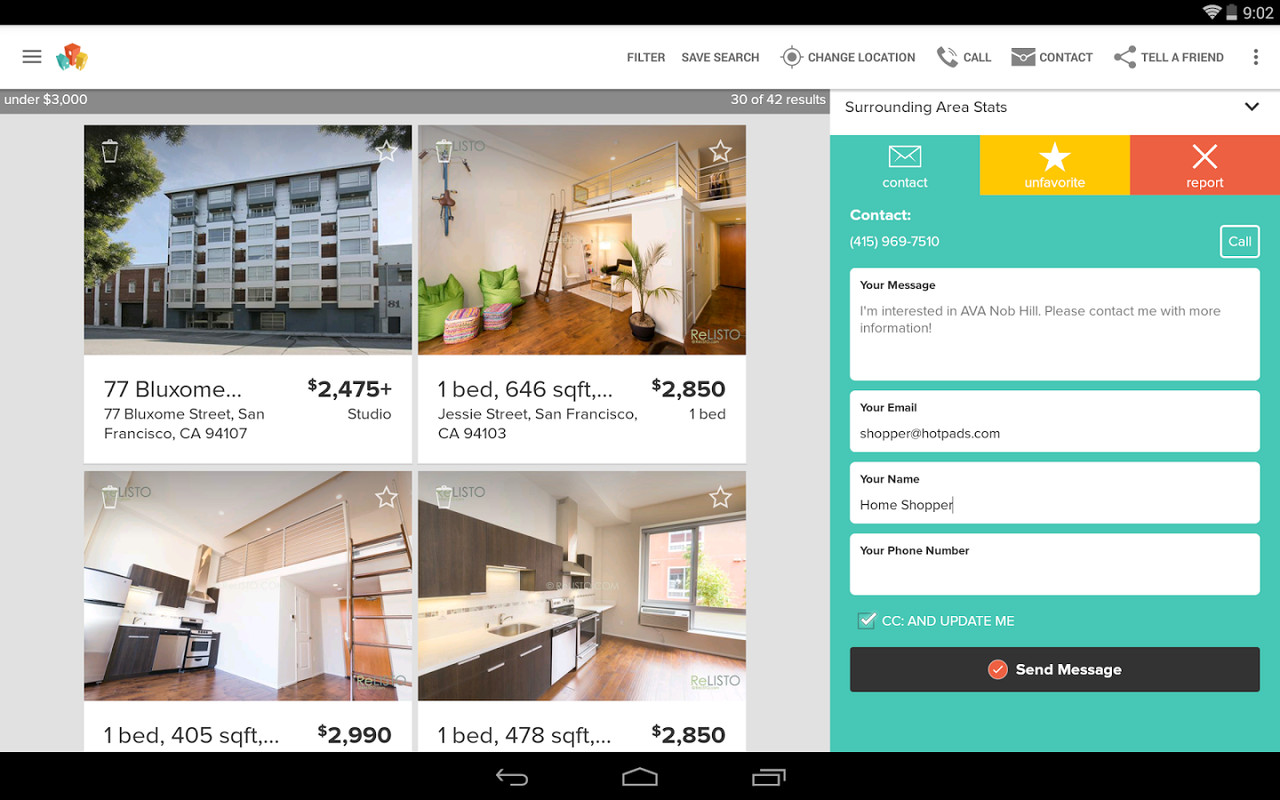This image depicts a detailed screenshot of a real estate and apartment website. In the upper left corner, there is a "List" button alongside an icon featuring green, red, and yellow colors. At the top right corner, a menu bar displays various options including "Filter", "Save Search", "Change Location", "Call Contact", "Tell a Friend". Directly below this menu, there is a dropdown box presenting "Surrounding Area Stats".

Three tabs with a teal background are also visible, labeled "Contact", "Unfavorite", and "Report". Below these tabs, there's a section designated for contacting via a displayed contact number and a button for placing a call. This section also includes fields for entering your message, email, name, and phone number, along with a "Send Message" button.

On the left side of the image, there are four square tiles showcasing pictures of apartments or homes. Each tile features bold black pricing on the right side, with additional property information listed below the images.